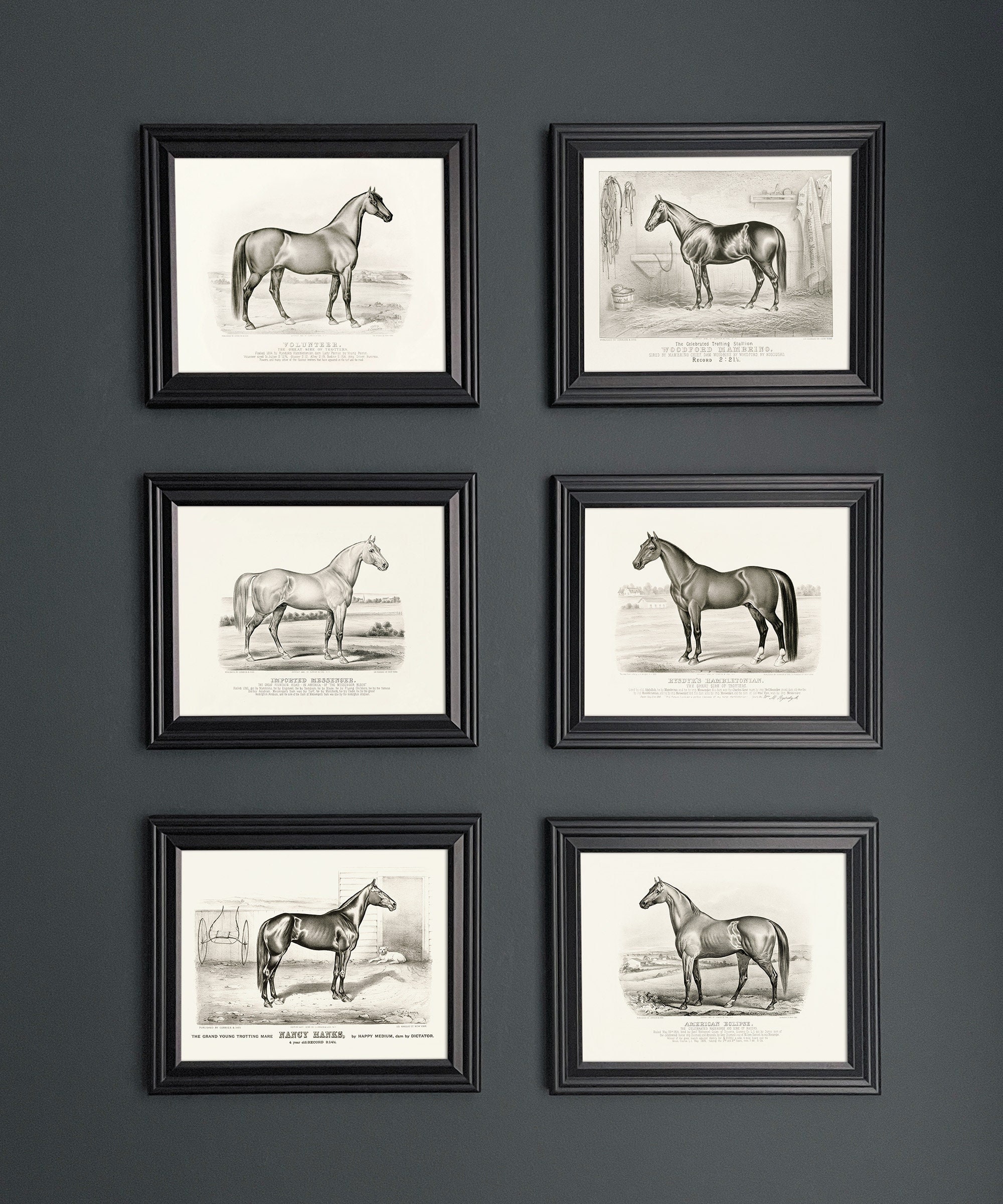This image depicts a photographic arrangement of six framed prints of horses, hung against a dark gray wall in a grid pattern with two columns and three rows. Each print is housed in a black rectangular frame. The left column features horses facing right, while the right column shows horses facing left. 

In the left column, the first row displays a gray horse, followed by a lighter gray horse in the same direction in the second row. The third row showcases a shiny, dark brown or black horse. These illustrations appear to be in various indoor and outdoor settings. Notably, the bottom-row horse in the left column stands in front of what seems to be a buggy set.

The right column begins with a horse in a stable environment, identifiable by hay, walls, a sink, and hanging clothes. The middle row features a black horse in a field, whereas the bottom row presents a light gray horse in another field.

All prints are set against a white backdrop, resembling illustrations or etchings. There is text beneath each image, but it is too small to be readable from this vantage point.